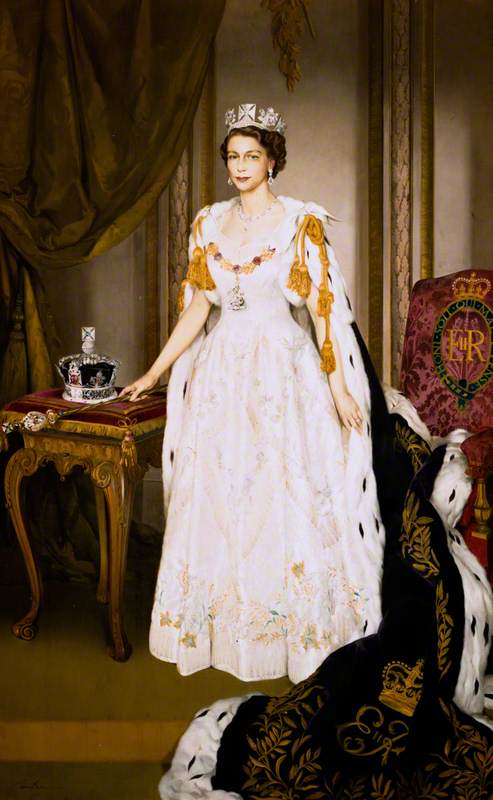This detailed artwork, whether a painting, colored drawing, or print, depicts a young Queen Elizabeth in regal attire. She stands center frame, gazing directly at the viewer, donned in a long, white floor-length gown with gold trim and gold-tassel epaulets on her shoulders. Her hair is short and brunette, crowned with a silver diadem featuring four curved crosses converging at the top. Queen Elizabeth accessorizes with elaborate, jewel-adorned silver earrings, a large necklace, and a pendant hanging from her gown's gold ropes.

Queen Elizabeth's right hand rests on a high wooden table, holding a scepter, with a full crown placed beside it. The backdrop includes dark drapes, adding to the opulent atmosphere. To her right, a chair with a purple back and embroidered Royal Crest with the letters "ER" is visible, further signifying her sovereignty. From her shoulders flows a richly decorated robe or cape, predominantly purple with a gold crown insignia above "ER," trimmed in white with narrow black elliptical shapes.

The room exudes an old-fashioned, ornate charm, with the green-floored setting enhancing the overall regality of the composition. This intricate portrayal captures the essence of Queen Elizabeth's royal presence, right down to the flowing gown and the red velvet chair adorned with a crest featuring a crown and green wreath to her left.